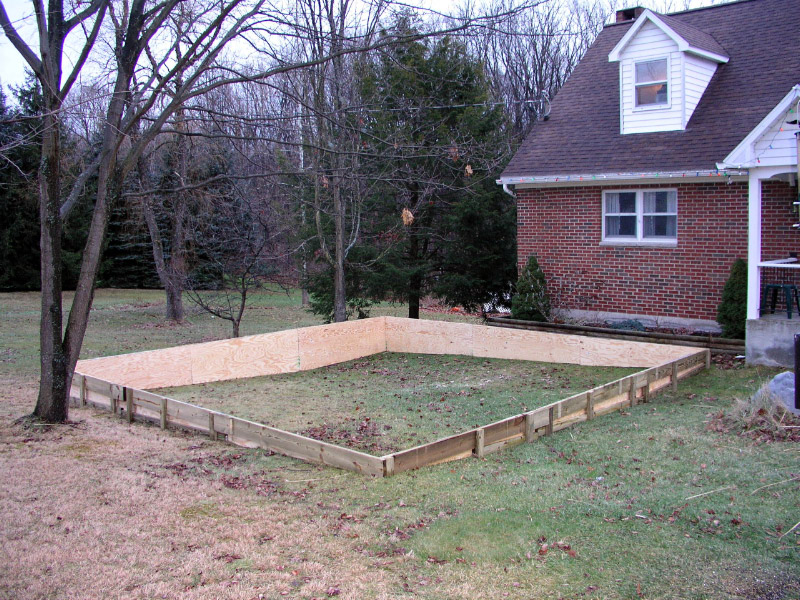In this outdoor image, it captures a winter or late fall scene in someone's yard, featuring a mix of green and browning grass speckled with fallen leaves and yard debris. Dominating the foreground is a wooden frame constructed from 2x4s and plywood, forming a large square on the ground. Adjacent to this wooden structure is a tree with branches that extend over the frame, hinting at uncertain future construction plans around it. Behind this setup stands a brick house, partially visible with red bricks and a dark brown roof. The house showcases two windows: one on the brick wall and another in the roof, where a light is illuminated. Additional details include unlit Christmas lights suspended near what appears to be a slightly out-of-frame front porch. Surrounding the scene are several trees, both evergreen and barren deciduous trees, further implying the winter season. The sky is clear, contributing to the overall calm and chilly atmosphere.